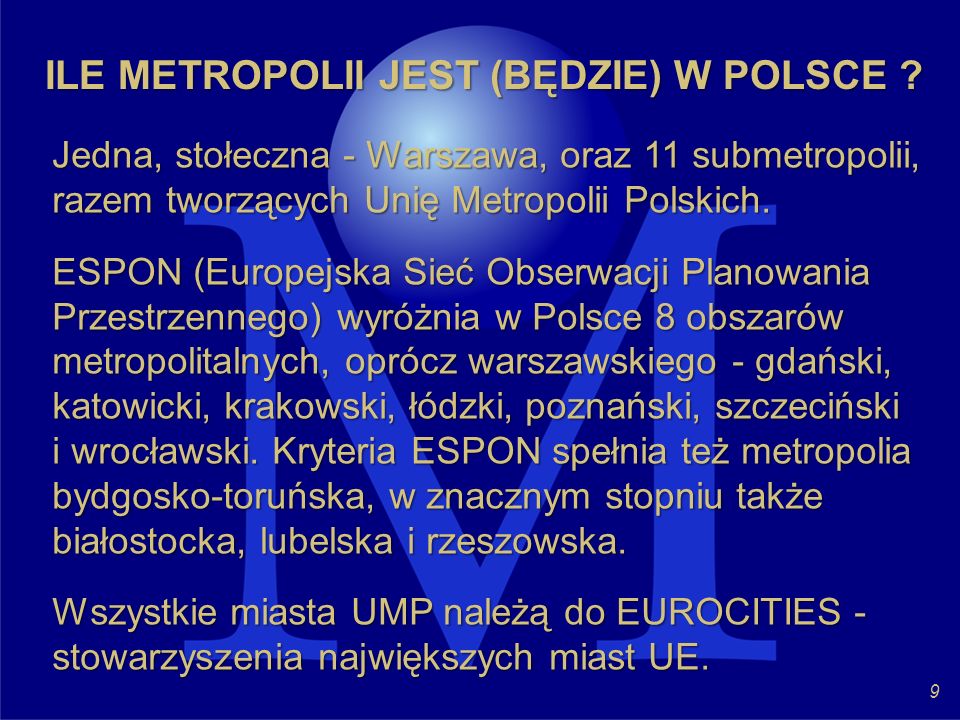The image appears to be slide number 9 from a larger presentation, indicated by the numeral in the lower right corner. The slide is slightly wider than it is tall and features a blue background with prominent gold or yellow text in Polish. Dominating the center is a large, faded letter "M" acting as a watermark, with what seems to be a three-dimensional white sphere or globe above it. The title and main text on the slide comprise multiple paragraphs, each listing words or phrases in Polish. The design elements and the presence of the watermark suggest an organized and professional presentation format.